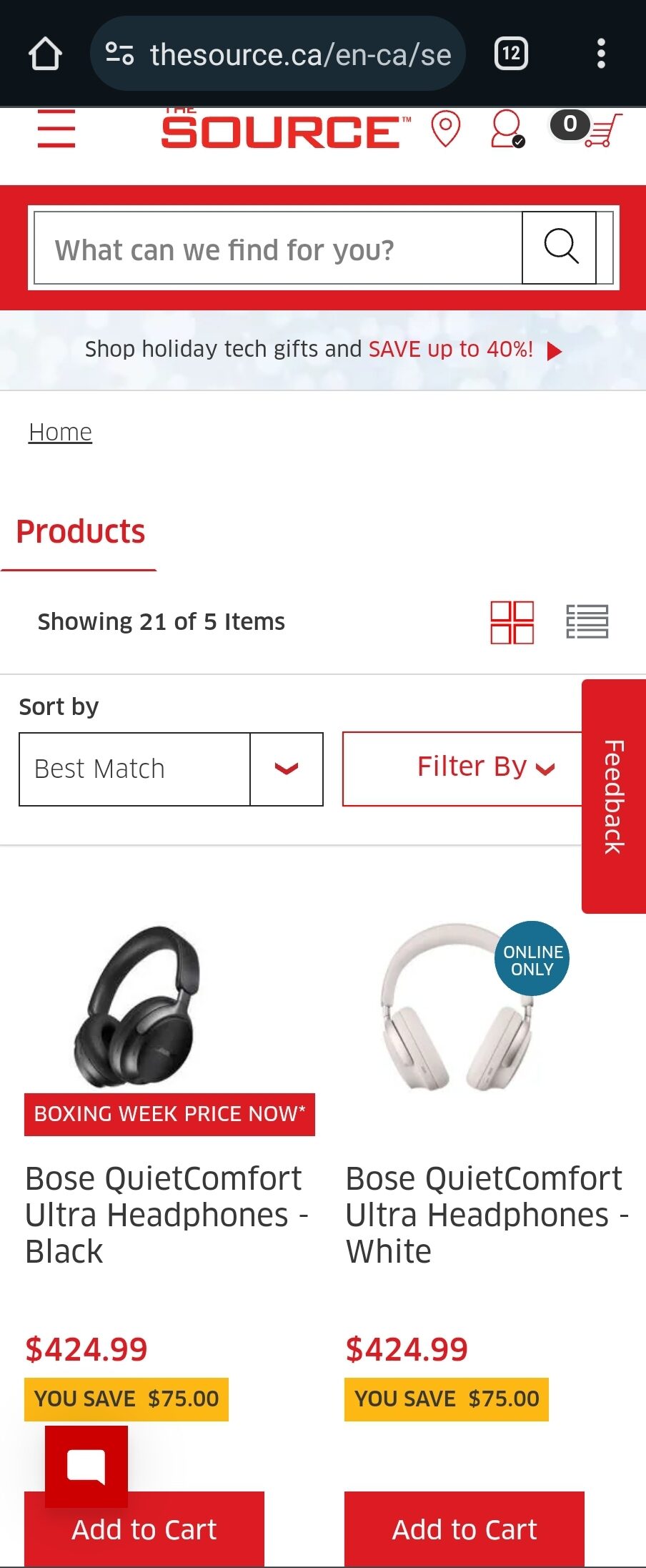The image depicts a webpage from "source.ca" with a distinct layout and multiple interactive elements. At the very top, a black border contains white text, alongside a home icon and a URL box displaying "source.ca/en-ca/se". Below this, the page features a white background showcasing three horizontal red lines stacked atop one another, and prominently displays "THE SOURCE" in large red capital letters.

Accompanying this header are several icons: a pinpoint icon indicating location services, a generic profile picture icon for account access, and a shopping cart icon featuring a black circle with the number "0" inside, suggesting an empty cart. A search bar with a red border sits beneath these elements, with placeholder text reading "What can we find for you?"

The segment immediately below includes a gray border and a promotional message proclaiming "Shop holiday tech gifts and save up to 40%". Following this, navigational text reads "Home" and "Product", indicating the current section, which is "Showing 21 of 5 items"—likely an error.

Further down, sorting options are presented with a drop-down menu labeled "Sort by" defaulting to "Best Match", and an additional "Filter by" drop-down menu. A red feedback button is also visible, inviting user interaction.

The lower part of the page visually features two pairs of headphones, displayed side by side—a black set and a white set—potentially as part of the holiday tech gifts promotion.